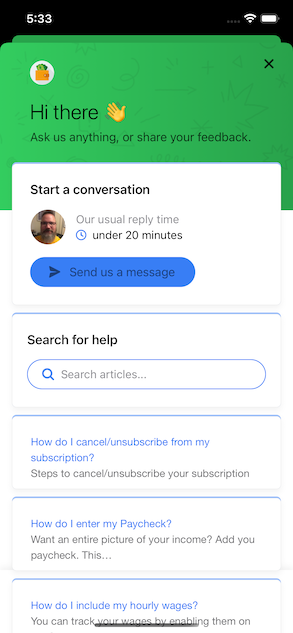The image displays a user interface, possibly on a tablet. The top section features a black bar with "5:33" on the left, a Wi-Fi symbol, and a full battery icon on the right. Below this, a vibrant green background contains a chat window with a message that reads, "Hi there! Ask us anything or share your feedback," accompanied by a waving hand emoji. An "X" is located in the upper right corner to close the chat.

Next, a prompt in darker green or black font reads, "Start a conversation. Our usual reply time: under 20 minutes." Beneath this is a blue button labeled "Send us a message." Below the button, there's a search feature framed by the text "Search for help" and "Search articles." This search bar includes a magnifying glass icon outlined in blue.

Following the search bar, a series of blue lines list FAQs with clickable questions, such as:
1. "How do I cancel/unsubscribe from my subscription?" in blue, followed by the gray text, "Steps to cancel/unsubscribe to your subscription."
2. "How do I enter my paycheck?" in blue, with accompanying black/gray text, "I want to enter the picture of your income. Add your paycheck..."
3. "How do I include my hourly wages?" in blue, with a description in black/gray, "You can track your wages by enabling them on..."

The interface is distinctly organized, using contrasting colors to differentiate between instructions, interactive buttons, and user input fields.